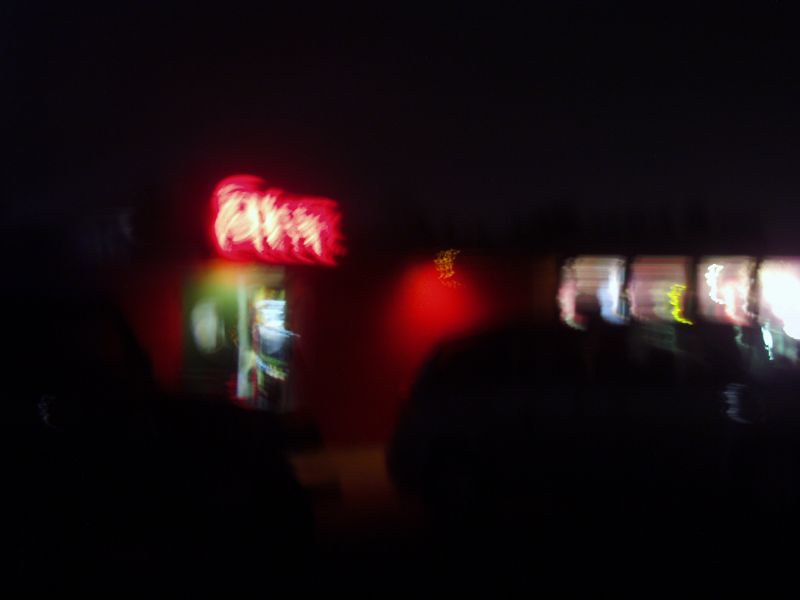The image presents a vibrant, neon-lit scene against a rectangular black background. Across the center, a medley of out-of-focus, brightly colored neon lights draw attention. Prominently, there's a red neon sign with indecipherable white text. Below it, a mix of green and blue neon, accented with white, adds more color to the composition. Central to the image is a neon depiction of a red rocket taking off, lending a dynamic element to the scene. To the right, four structures are adorned with an array of neon signs. The farthest right building glows with an intense, glaring white light. Next to it, another structure shines predominantly white, while the third building features a striking yellow streak descending its facade. The fourth structure on the left appears to have a dark entrance, adding depth to the bustling, illuminated cityscape.